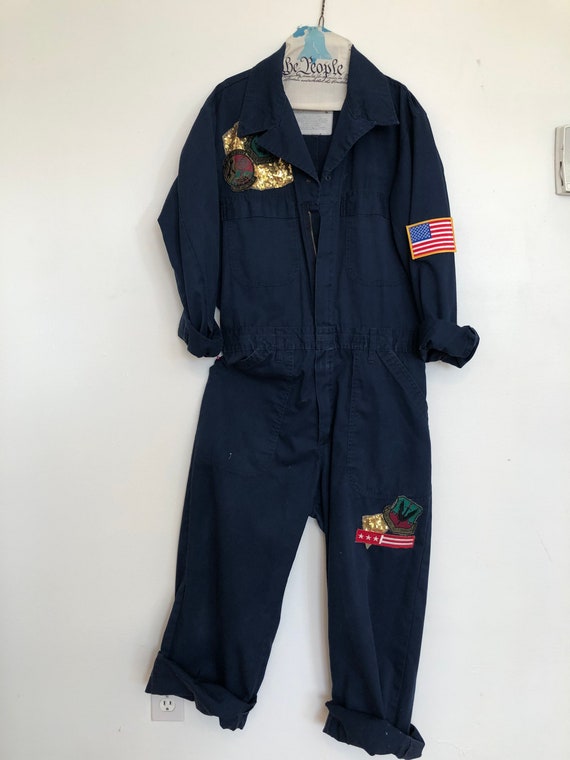The image depicts a dark navy blue military uniform hanging on a wire hanger against a white wall, likely inside an apartment. The uniform consists of a jumpsuit or coverall with a partially open zip-up front. The cuffs of both the pants and the shirt are rolled up. On the left sleeve, there is a prominent patch of the American flag. The upper right chest features some bright golden patches, possibly reflecting light from the camera, and depicting a circle with a tool. Over the left knee, there is another patch featuring a red and white band with three white stars. The wire hanger has a tissue paper covering, which appears to have an advertisement, possibly saying "We the People" or similar text. In the background, there is a visible thermostat control and an electrical outlet on the wall, providing context to the indoor setting.